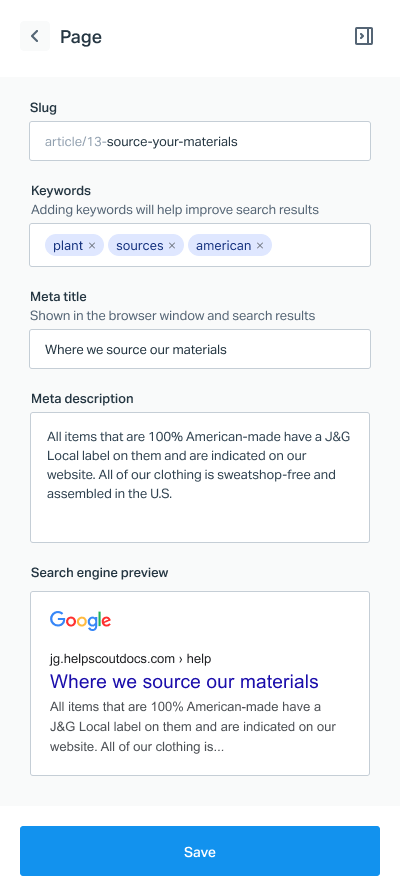The website features a clean white background with a well-organized interface. On this specific page, there are navigational elements including a left arrow, a white arrow, and a square icon. The URL slug reads: "article/13-source-your-materials."

The page underlines the importance of adding keywords, noting that they will help improve search results. There are three gray ovals in blue, representing some form of visual indicator or selection tool.

The content emphasizes plant sources within the American context and includes metadata for SEO purposes. The meta title, which appears in the browser window and search results, is: "Where we source our materials."

The meta description provides additional information about the sourcing process and includes a preview of how the page will look on search engines, specifically showing an example URL: "Google JG.help scout.docs.com."

Further down, there is a right arrow labeled "Help" in blue. The main content of the page reiterates the company's commitment to sourcing materials from the United States, stating: "All items that are 100% American made have a JNG local label on them and are indicated on our website. All of our clothing is..."

Finally, there is a blue rectangle button at the bottom of the page with the options "Save" and "Wipe."